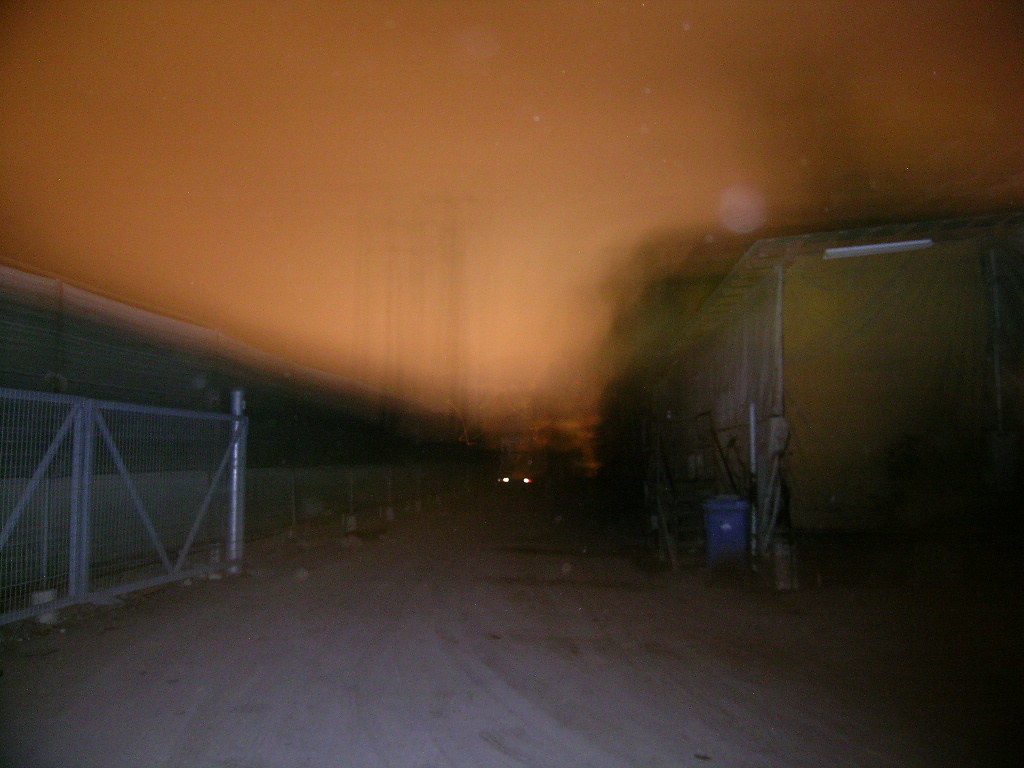This color photograph, possibly digitally altered, presents a night or near-night scene with a strikingly ominous, burnt orange sky that dominates the upper section. The image is somewhat blurry, adding to the eerie atmosphere. In the foreground, a road with a gravelly or sandy texture stretches out, appearing grayish under the surreal sky. On the left side of the photo, a large silver metal gate stands open. To the right, there is a green trailer or building, partially obscured by darkness, with a large blue garbage can placed nearby. The middle of the image features two bright, white lights that might be headlights of an approaching vehicle, though their ambiguous, eye-like appearance could suggest an animal or another creature. The scene is dotted with indistinct shapes and shadows, enhancing the enigmatic quality of the photograph.